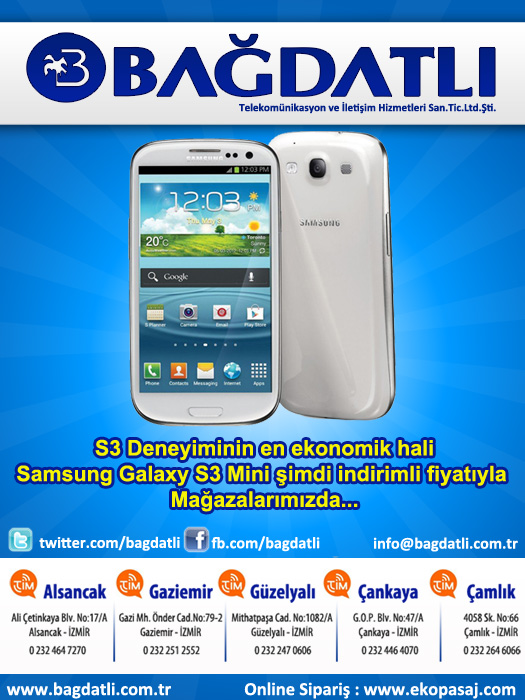The image is a detailed advertisement for Baghdadli, a technology retailer potentially based in Turkey. The central focus of the advertisement is the promotion of the Samsung Galaxy S3 mini, prominently featuring both the front and back views of a white Samsung Galaxy S3 phone. The front screen of the phone displays details like the time (3 minutes past 12), temperature (20 degrees), and various app icons including Google. The advertisement predominantly uses a blue and white color scheme, with accent colors in orange and yellow for certain text elements. At the top, the name Baghdadli is clearly displayed. Additional elements include social media links and handles for platforms such as Twitter and Facebook, and multiple web addresses like www.Baghdadli.com.tr and www.ecoparski.com. The bottom section of the advertisement lists several store locations and contact information alongside a logo that resembles a dog with a bee.